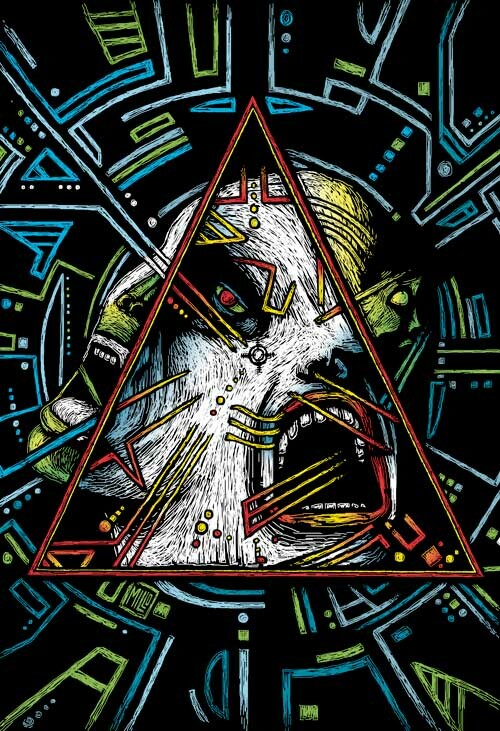The image features a striking and complex design set against a black background. At its center is a vertical rectangle showcasing a prominent triangle outlined in yellow and red. Within the triangle are two overlapping heads, both with white, fur-like textures. The head on the right appears to be mostly white with a partially open mouth exposing white teeth, a green nose, and a green chin. Its eye is characterized by a green sclera and a red iris. The left head, slightly smaller, is oriented upwards and leftwards, seemingly without eyes, but with visible yellow hair that extends out of the top right of the triangle.

The triangle itself contains intricate geometric shapes including small yellow circles and a series of V shapes. Yellow lines outline parts of the triangle, which shift into orange where they converge. Surrounding the triangle is a circular design resembling a maze with numerous symbols, geometric figures, lines, and dots extending within its borders. Predominant colors in the circular design include white, blue, and green. The base of the triangle features a possible signature that resembles the name "Milo," adding a final touch to this intricate and layered graphic.